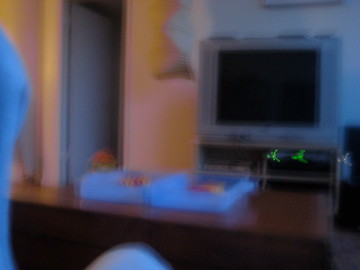In this low-resolution and extremely blurry image, one can vaguely discern a living room setting. Dominating the scene is an old, possibly vintage television, accompanied by a coffee table positioned in front of it. At the edge of the frame, there appears to be part of a couch. Despite the lack of clarity, a couple of white trays are visible on the coffee table, though the contents within them remain indistinguishable due to the image quality. This scene offers a nostalgic glimpse into a home interior, albeit shrouded in mystery and pixelation.